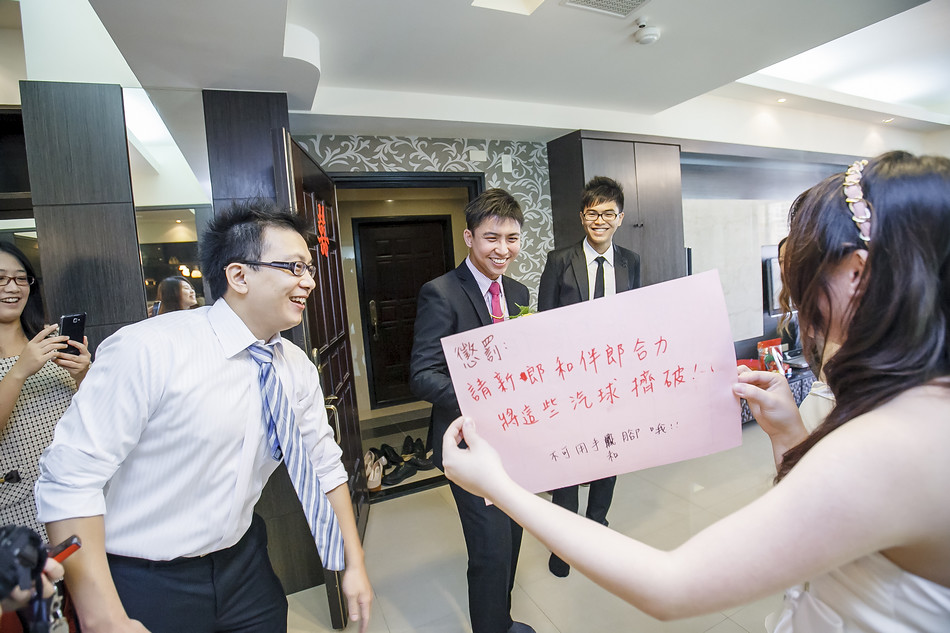In the image, a vibrant scene unfolds inside a luxurious indoor setting, possibly a hotel or an upscale event venue. Central to the composition, a young woman dressed in a white, shoulderless dress stands to the right, holding a pink sign with red, handwritten Chinese characters. The group around her appears captivated by the sign, with three young men on her left, dressed in formal shirts and ties, two of whom are wearing suits and glasses. They are engaged, smiling, and laughing as they look at the sign, evoking a sense of communal enjoyment. On the far left, another young woman captures the moment on her phone, further emphasizing the lively and joyous atmosphere of the gathering. The background reveals tiles on the floor, elegant wallpaper, windows, and a door, contributing to the clean and sophisticated ambiance of the event.